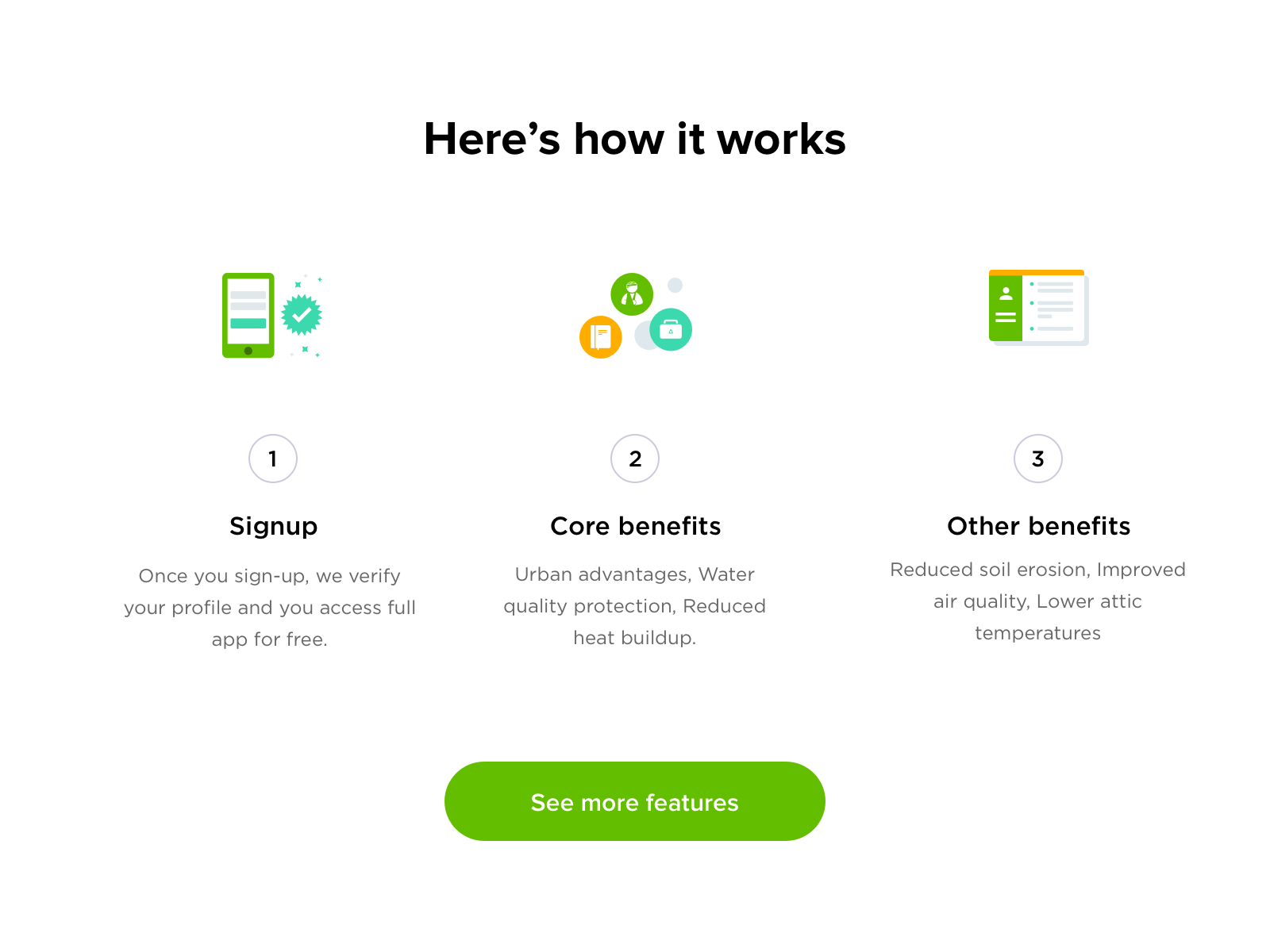Screenshot of a minimalist web page with a clean, white background. The page is organized with three small icons and accompanying text prominently displayed. The header at the top of the page is in bold black text, reading "Here's How It Works."

1. Starting on the left, there is an icon of a phone with a blue line towards the bottom and a check mark beside it. Below the icon, a circled number "1" is labeled. The bolded text "Sign Up" follows, with a smaller, non-bolded description: "Once you sign up, we verify your profile and you access full app for free."

2. Centrally located, a cluster of three icons—a doctor, a briefcase, and a notebook—sits above the circled number "2." The bolded label "Core Benefits" is followed by the smaller text: "Urban advantages, water quality protection, reduced heat buildup."

3. On the right-hand side, an icon of an ID card is placed above the circled number "3." The bolded text "Other Benefits" is followed by the smaller description: "Reduced soil erosion, improved air quality, lower attic temperatures."

At the bottom center of the page, a green button labeled "See More Features" invites further exploration.